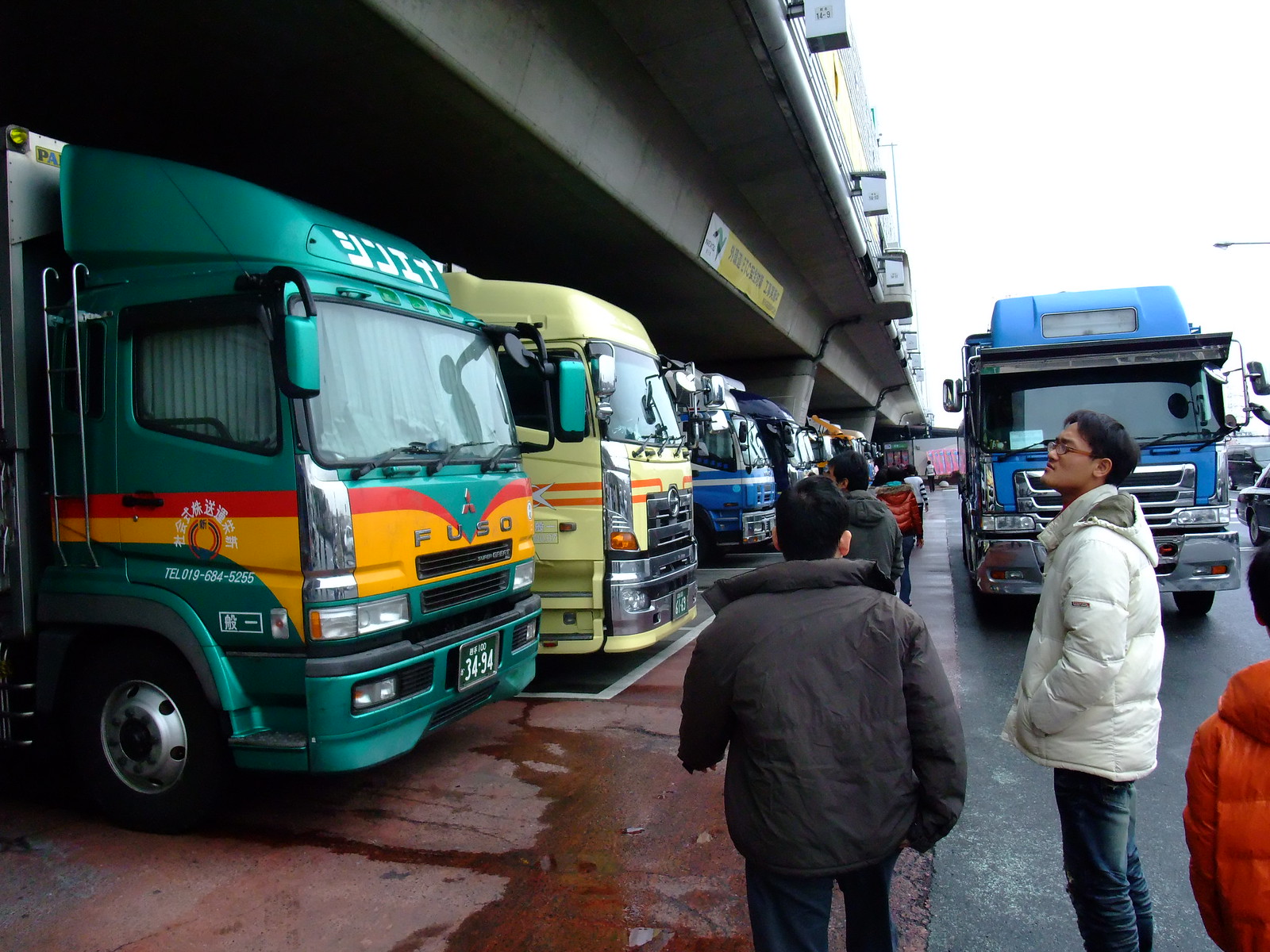The image captures a bustling scene within a multi-level parking garage in an Asian country, possibly Japan, China, or the Philippines, given the distinctive Oriental lettering on the vehicles. The high-rise concrete structure, marked by a white and yellow sign on top, houses a fleet of brightly colored semi-trucks and RV-like buses. In the foreground, a shiny green RV with curtains in the front windows, adorned with red and yellow borders, stands out. It is complemented by a line of other vividly colored vehicles, including a pale yellow RV with orange stripes, blue and purple trucks, an orange truck, an aqua Fuso truck with Japanese or Chinese lettering, and another yellow truck.

Amidst them, four people mill about—one wearing a brown jacket and black pants, another in a beige puffy jacket and blue jeans, with a glimpse of a person in a red coat. The road is a smooth black tar, contrasting with the brownish-red tiled or cement floor of the parking bays. The scene appears to follow a recent rain shower, given the wet surface reflections, adding a fresh, vibrant feel to the image. The trucks are parked in a well-lit, extensive structure designed to shelter them from the weather, creating an organized and vibrant snapshot of a bustling vehicle hub.